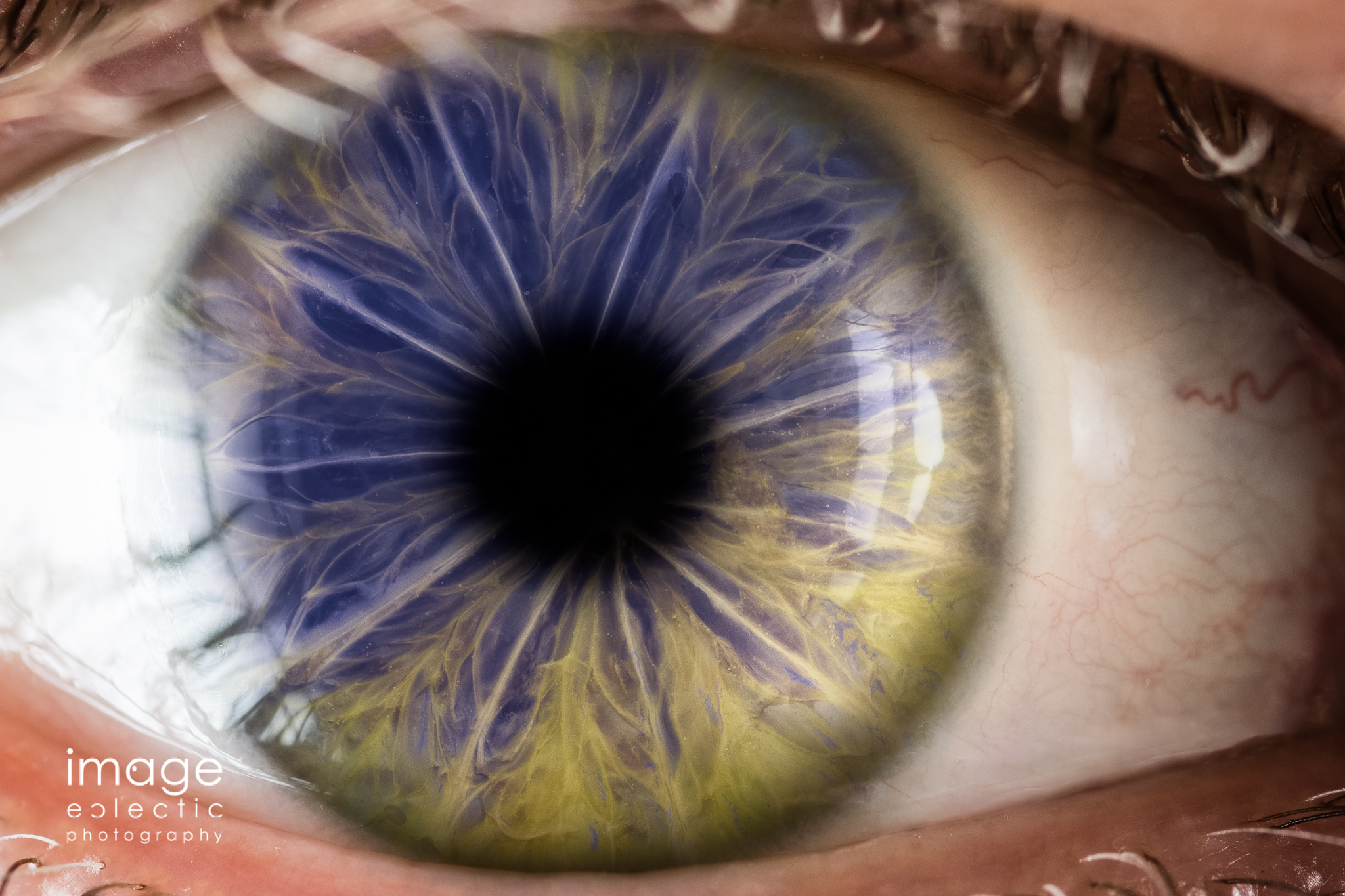This image, credited to a photographer with the stylized logo "Image Eclectic Photography" (featuring a backwards "C" in "Eclectic"), is a highly detailed, extreme close-up of a Caucasian person’s eye. The photo, in full color, captures the intricate details of the eye, including separated dark eyelashes and visible veins within the white area of the eye on the right. The main focus is on the pupil and the iris, with the iris exhibiting an unusual and digitally manipulated marbled effect, reminiscent of toy marbles. The iris features a deep royal blue at the top, transitioning into a golden yellow at the bottom, further accentuated by marbled patterns and starburst-like white highlights around the pupil. The reflection of what appears to be an open window behind the photographer is also visible, adding to the realistic shading and reflections of the image. The upper eyelid is partially visible with some eyelashes, while the lower lid edges into the frame, making for an engaging and almost surreal close-up of the human eye.